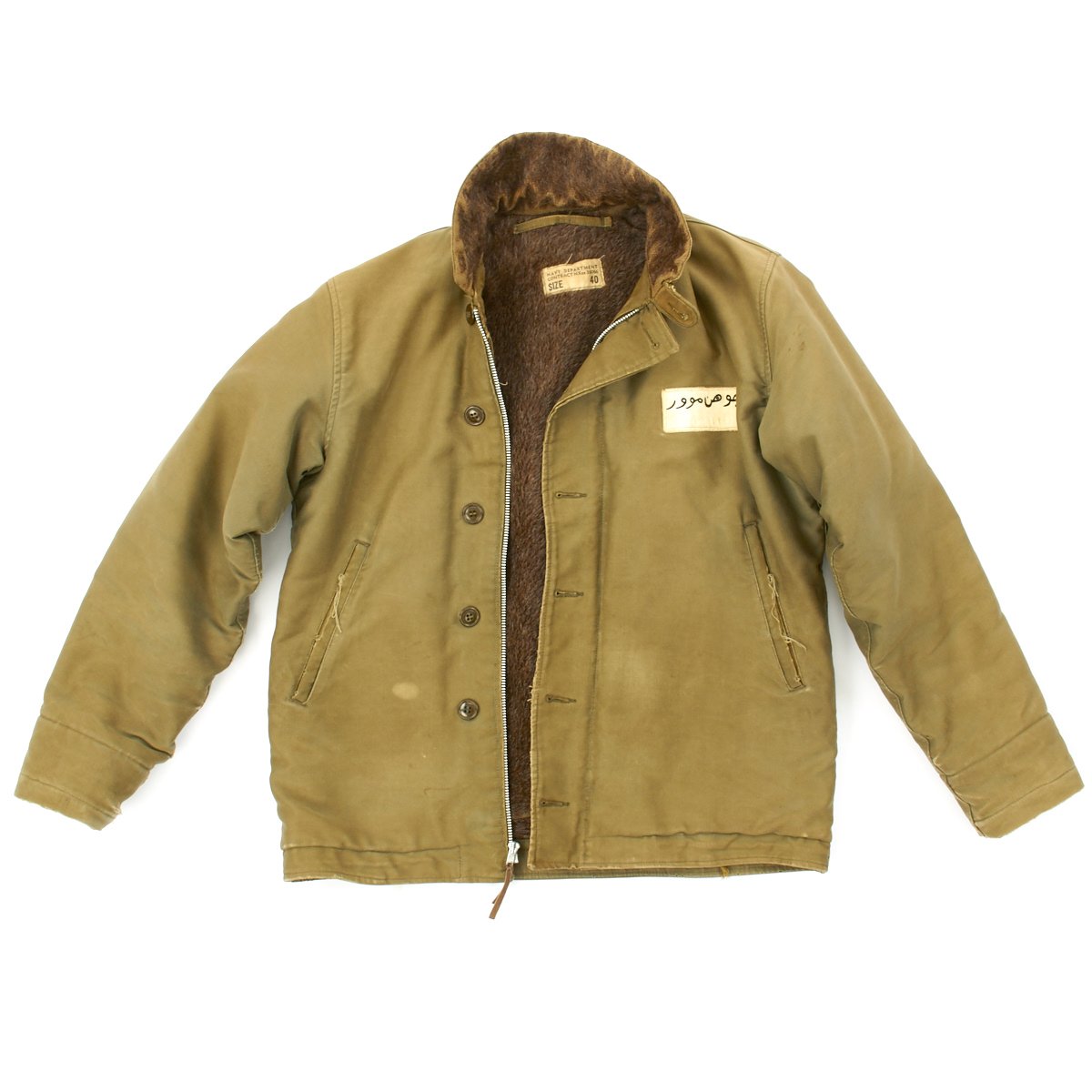This photograph features a long-sleeved jacket displayed on a plain white background, emphasizing the garment itself. The jacket is an olive green to tan color on the exterior, with a luxurious fur or wool lining intended for warmth. The interior, including the fuzzy collar, is a rich brown. A silver zipper runs up the front beneath a panel with six brown buttons, three on each side. The jacket includes functional pockets on both the left and right sides and is designed without a hood, but the neck area can be fastened closed with a button. A tag on the upper right, possibly in Arabic, and another tag inside indicating the size, whether it's 40 or 49, adds further detail to the garment.